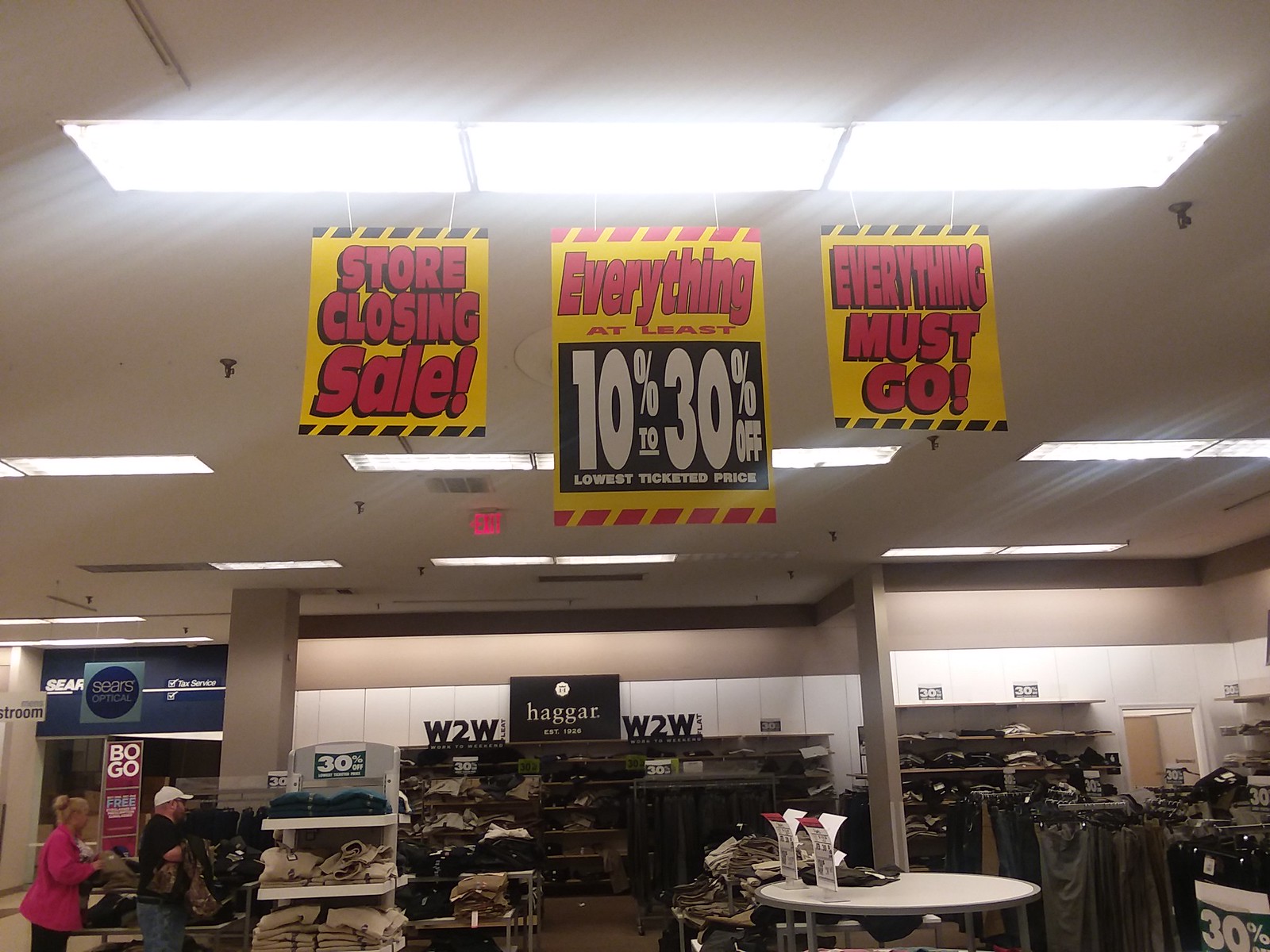The image depicts the interior of a department store undergoing a "Store Closing Sale." The scene features various racks of clothing and strategically placed merchandise. In the foreground, there are multiple racks filled with diverse apparel, including shoes. Towards the back wall, folded clothes are visible, likely including jeans and jackets on the left side. Hanging from the white ceiling with three prominent lights are vibrant signs that stand out with their bright yellow and red colors. The middle sign declares, "Everything at least 10% to 30% off, lowest ticketed price." The sign on the left announces, "Store Closing Sale," and the one on the right emphasizes, "Everything must go." There are also visible labels like "Hager" and "W2W" in the background. On the left side of the photo, a woman in a purple or pink dress and a man wearing a white hat along with a black shirt are engaged in shopping. The store's light beige walls and overall ambiance suggest an intense clearance event, with all items marked for urgent sale.